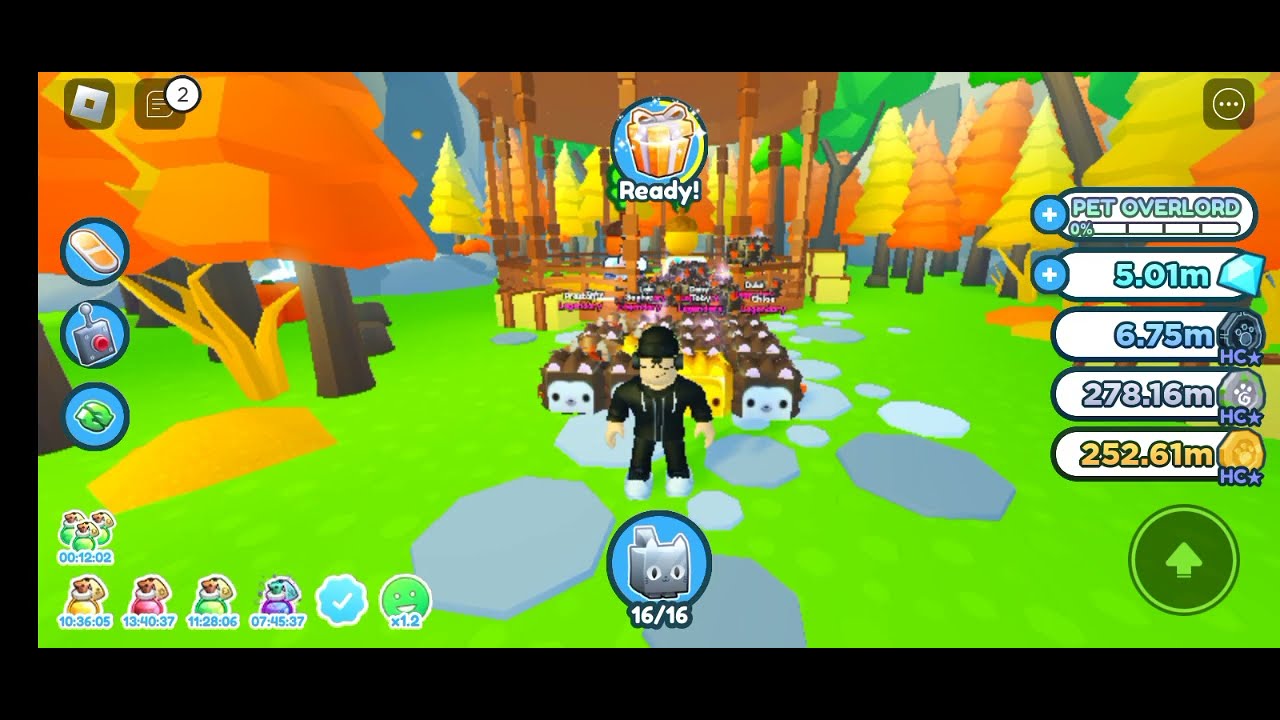This vibrant and detailed screenshot from a video game features an outdoor ground area covered with lush green grass, accentuated by numerous trees in autumnal shades of orange, yellow, and green. In the center of the scene stands a humanoid character dressed entirely in black, complete with a shirt, pants, hat, over-the-ear headphones, and black glasses, exuding a stylish and somewhat enigmatic presence. Directly behind this figure, a group of cube-shaped cat heads, reminiscent of animated characters, adds a quirky and playful element to the scene. 

The background showcases a wooden building structure, lending a rustic touch to the environment. The periphery of the screen is lined with various game icons and statistics; on the right side, you can see measurements such as "5.01 M," suggesting some form of score or resource tally. The top of the screen features a banner with the word "READY," flanked by an opening present icon, while the bottom displays an icon indicating "16 of 16" cats. Additionally, notable icons like a band-aid and other interactive buttons help players navigate and manage their game. Finally, black horizontal strips at the top and bottom of the image frame the screenshot, focusing attention on the colorful and dynamic scene within.